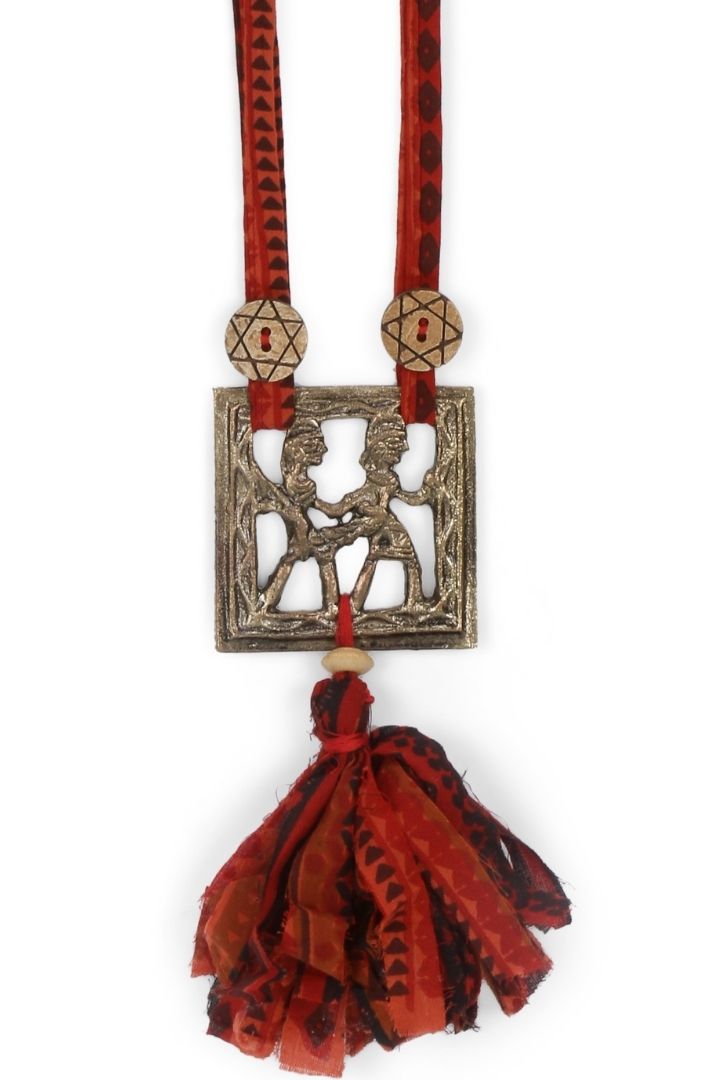This photograph captures an intricate and possibly antique necklace or medallion with profound details. At its center lies a square metallic piece, possibly made of silver or bronze, featuring a carved outline that encloses two figures, which appear to be walking to the right—potentially a depiction of Native American subjects. The center is hollow except for the thin metallic outline and the figures within. Extending upwards from the medallion are two red ribbons adorned with black triangular decorations which feature circular star-like buttons that resemble Jewish stars. These ribbons are fastened through the top of the medallion and continue downwards beneath it, where they culminate in more red fabric. This fabric is bunched up in a manner reminiscent of a large pom-pom or tassel, and it is threaded through a tan bead positioned at the top of this section. The overall design showcases a combination of old-world craftsmanship and cultural symbolism, highlighted by the detailed metallic carvings and the vibrant red ribbons.